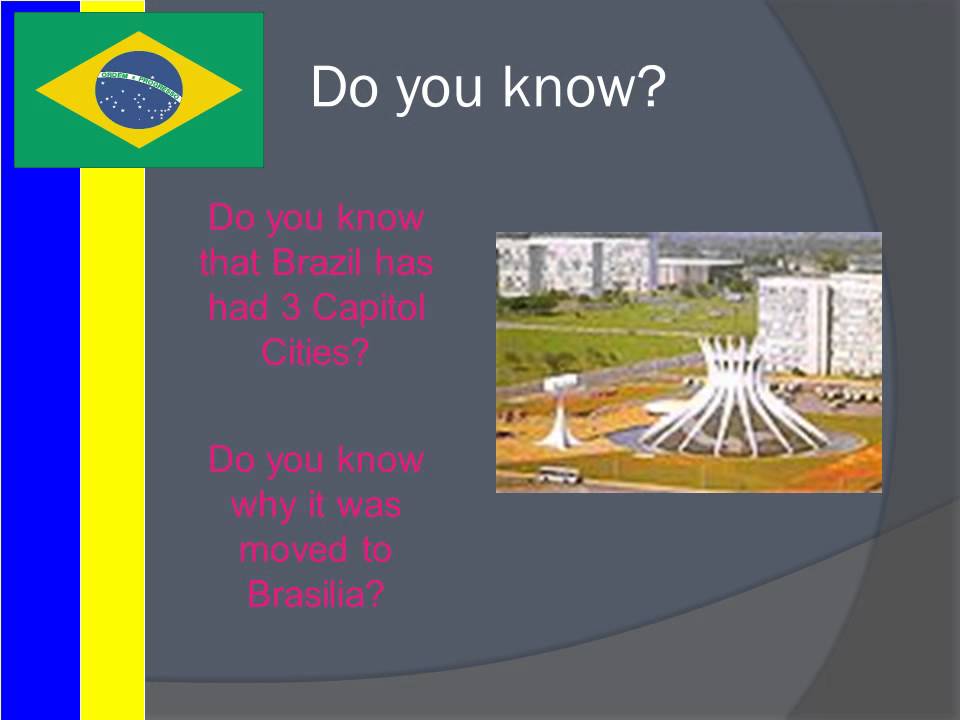This horizontal web image, potentially used as part of a web page, features an abstract design with three different shades of gray forming the main background. On the left side, vibrant neon blue and neon yellow strips add a striking contrast. At the top left corner, a green rectangle contains a yellow diamond and a blue circle, with a white curved line cutting across the circle and green text displayed on it.

Large white text at the top of the image reads, "Do you know?". Beneath this, on the gray portion of the background to the left, is a bright pink message: "Do you know that Brazil has had three capital cities? Do you know why it was moved to Brasília?".

To the right of this text, an inset and very pixelated image shows a white spiral structure resembling a dome with a crown, surrounded by greenery and tall white buildings, indicative of a cityscape. The secondary image includes hues of white, green, and orange, set against a gray sky.